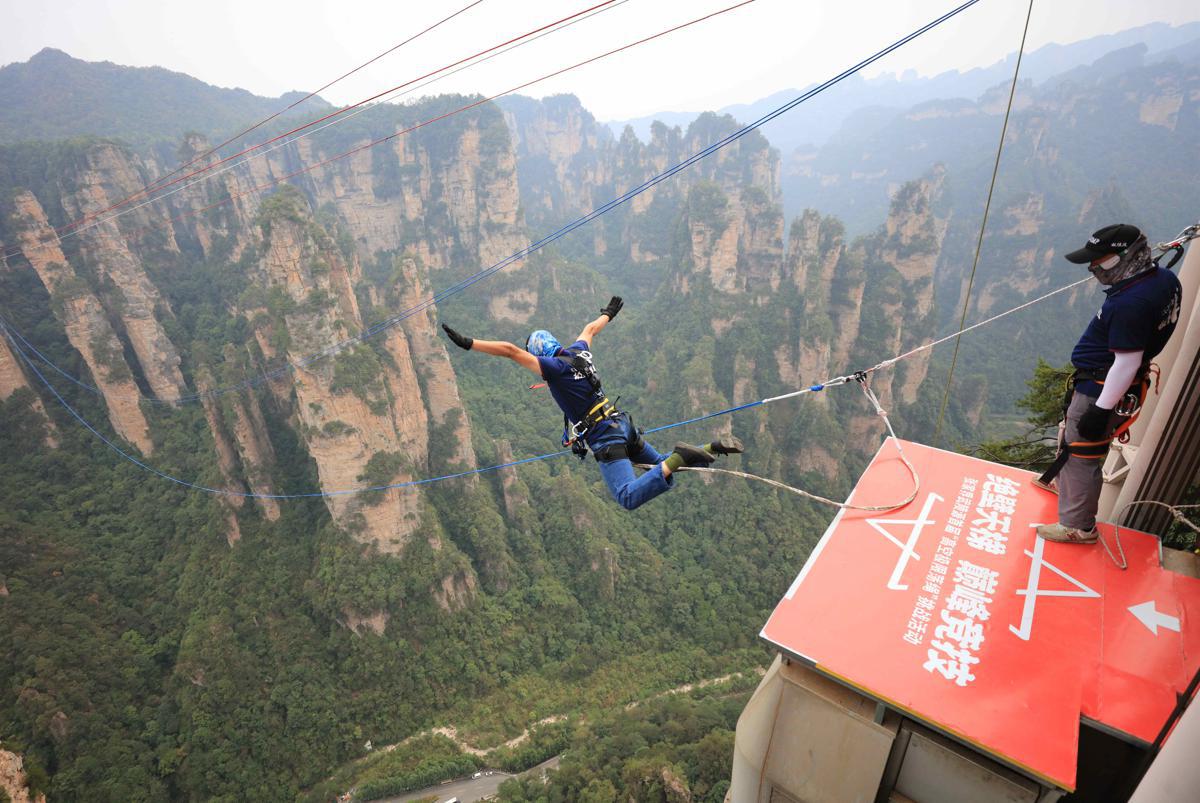In this captivating color photograph, a man is captured mid-bungee jump against a breathtaking, hazy mountainous backdrop. The scene is set on a bright orange platform adorned with Asian script and a white mountain symbol, suggesting an Asian locale. The jumper, sporting blue jeans, a black vest, a helmet, and a harness, has just leapt off the platform with his arms extended and legs trailing behind. Suspended above a deep ravine, he is tethered by a bungee cord that blends with a web of multi-colored ropes—white, red, and blue—stretching across the valley to distant, steep cliffs.

In the background, the mountain's sheer rock faces interspersed with patches of green vegetation and climbing trees add to the dramatic scenery. A second man stands on the platform, watching the jumper's daring dive. He is dressed in a dark blue shirt, gray pants, black gloves, and a black hat with a visor, and his face is covered by a mask. The visibility is low due to the foggy, cloudy atmosphere, contributing to the sense of both adventure and mystery enveloping the participants and their awe-inspiring surroundings.